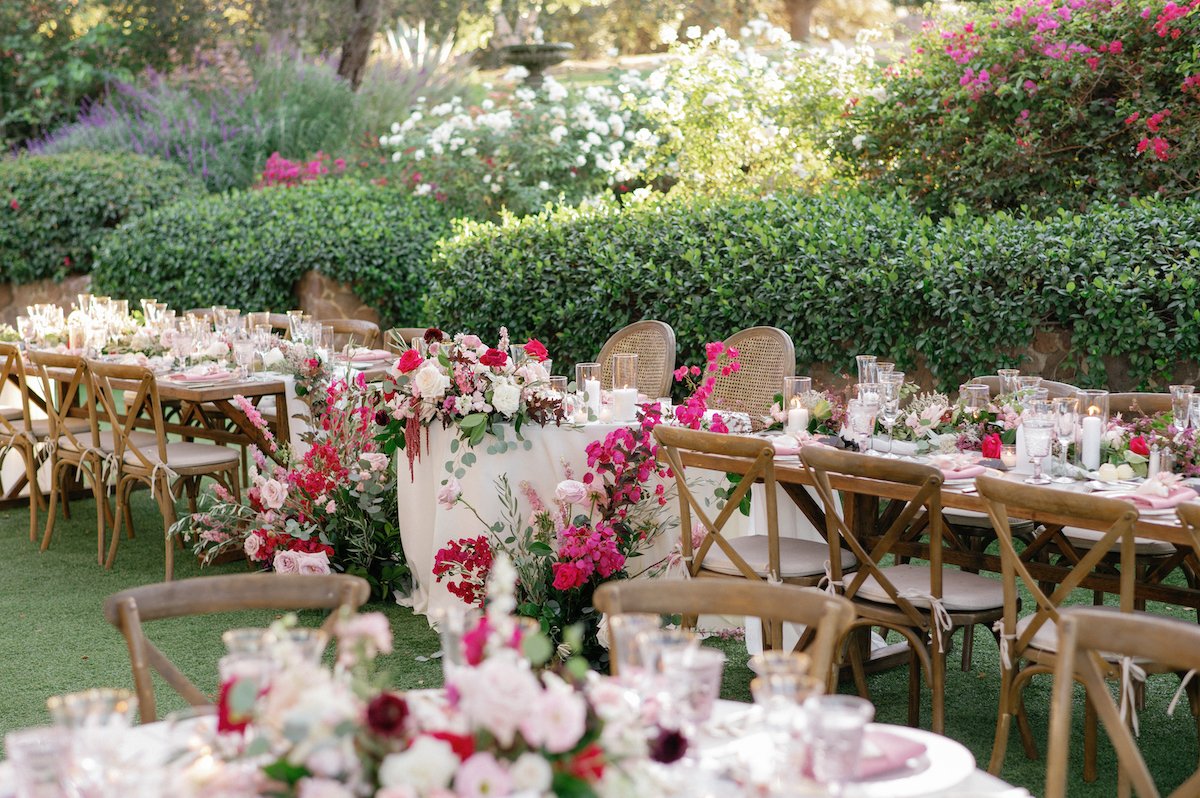A beautifully detailed photograph capturing an exquisite outdoor banquet, likely set for a wedding, nestled within a lush, well-maintained garden. The setting showcases a harmonious blend of elegant decorations and nature's splendor. At the center of attention is a grand, long table flanked by neatly arranged chairs, all adorned with pristine glassware, cutlery, and candles. The tables are graced with crystal vases holding flowers in various shades of pink, red, and white, perfectly matching the surrounding decor. A round table in the forefront and a specially designated table with two larger chairs suggest preparations for an intimate celebration. The garden's edge is adorned with colorful blooms—vibrant reds, whites, fuchsias, purples, and pinks—providing a private and serene backdrop. Every detail appears meticulously arranged, ready to welcome guests to this enchanting venue.